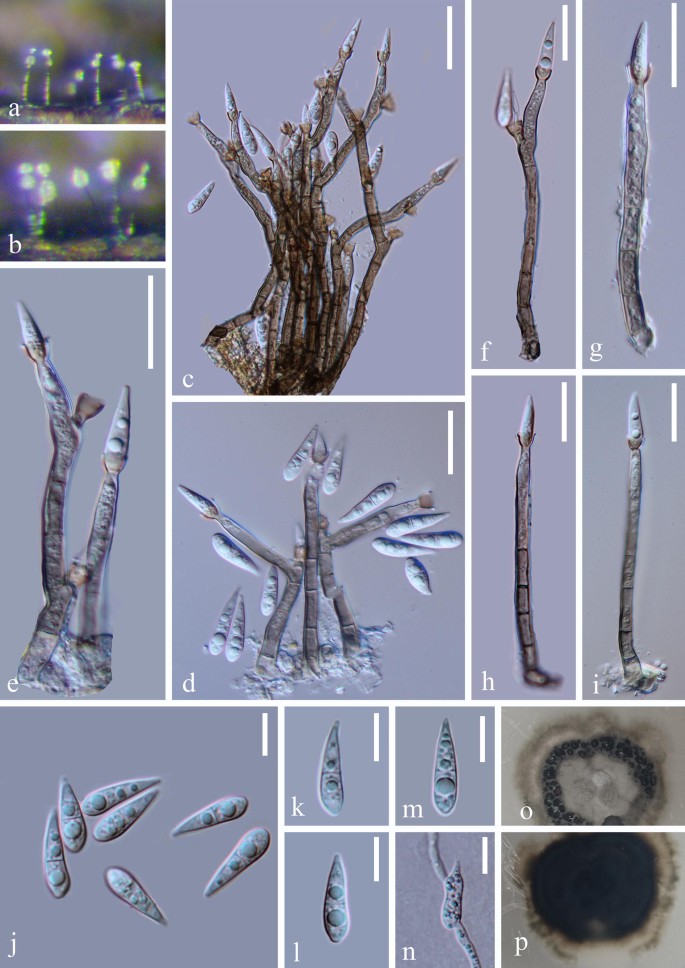The image is a collage consisting of micrographs divided into 16 labeled sections, from A to P. Each section features detailed, zoomed-in views of microscopic entities that resemble organelles or plant-like structures. Sections A and B at the top display lit-up end segments with a mix of brown and green hues, showing bulbous, stem-like structures that appear almost translucent. The middle sections, C to N, all sit against a gray background and display varying arrangements of these microscopic entities, with C focusing on a clump and F to I showcasing single strands. J to N feature structures that resemble seed pods, marked by their distinct shape. Sections O and P at the bottom right are distinguished by a dark gray circular ring in the center. The overall layout includes varying shapes and sizes of rectangles and squares, with clear delineations and a mixture of lighter and darker gray tones, giving the appearance of an organized array of microbial or cellular forms.